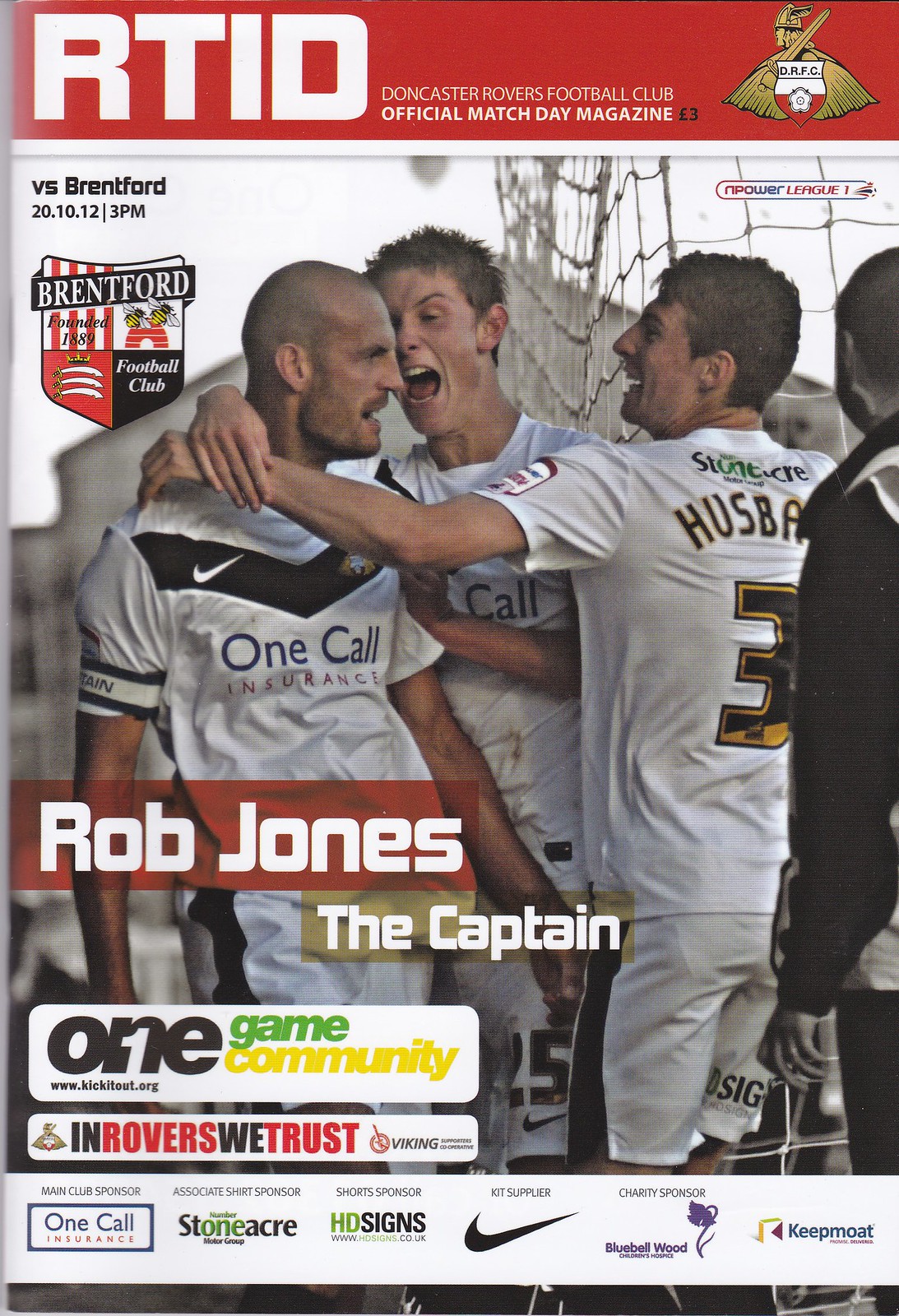The image depicts the cover of the official Doncaster Rovers Football Club Match Day Magazine, priced at 3 British pounds. At the top of the cover, a prominent red banner features the letters "RTID" in large white font. Below this, the magazine title is written in smaller white text: "Doncaster Rovers Football Club Official Match Day Magazine." In the upper right corner, there is an emblem of a gold Viking wielding a sword, set against a shield with "DRFC" inscribed.

The center of the cover showcases a vibrant color image of three soccer players in white uniforms with black accents, huddling closely in a celebratory embrace. Overlaying the leftmost player is a red stripe that reads "Rob Jones," followed by "The Captain" in smaller text beneath it. On the left side of the image, above the players' heads, is a crest featuring a shield with red, white, and black elements, marked with "Brentford, founded in 1889," indicating the opposing team. The crest includes three swords and two Bs, symbolizing Brentford Football Club.

Toward the bottom left of the cover, two white textual bars appear: the upper bar reads "One Game Community," and the lower bar states "In Rovers We Trust." At the bottom of the page, a horizontal white strip contains six sponsor logos, including recognizable brands such as Nike and Bluebell Wood Children's Hospice, among others, providing a comprehensive representation of the magazine's collaborative supporters.